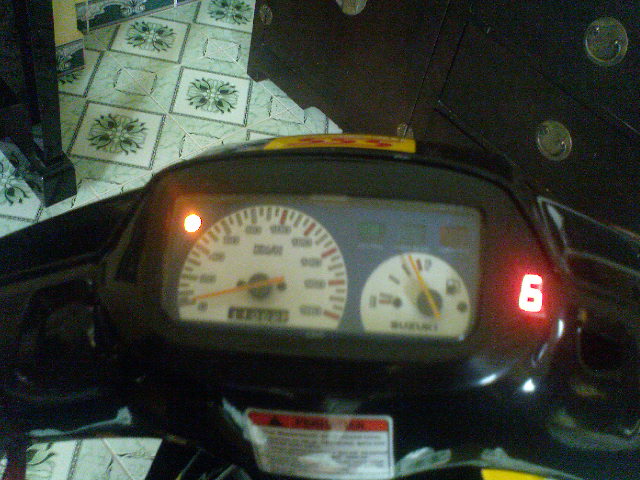This photograph captures the control display panel of a scooter, prominently featuring two rotating dials. The panel itself is encased in black plastic with a roughly rectangular shape and has curved black plastic handles extending out to both the left and right. The display shows two round dials: the left one indicating speed, and the right one showing the fuel level, which is almost full according to the orange needle. A glowing red indicator light is visible in the upper left corner of the display, and a lit number '6' is present on the right side of the screen.

The background reveals a detailed setting, with gray tiled floors adorned with white diamonds featuring a square floral pattern in their centers. In the upper left corner, a black metal table leg is visible, while the upper right corner shows the edge of a dark brown wooden dresser with elegant gold ring handle pulls. These elements provide a contrasting backdrop to the scooter’s display panel, focusing attention on the scooter's controls while offering context to its surroundings.